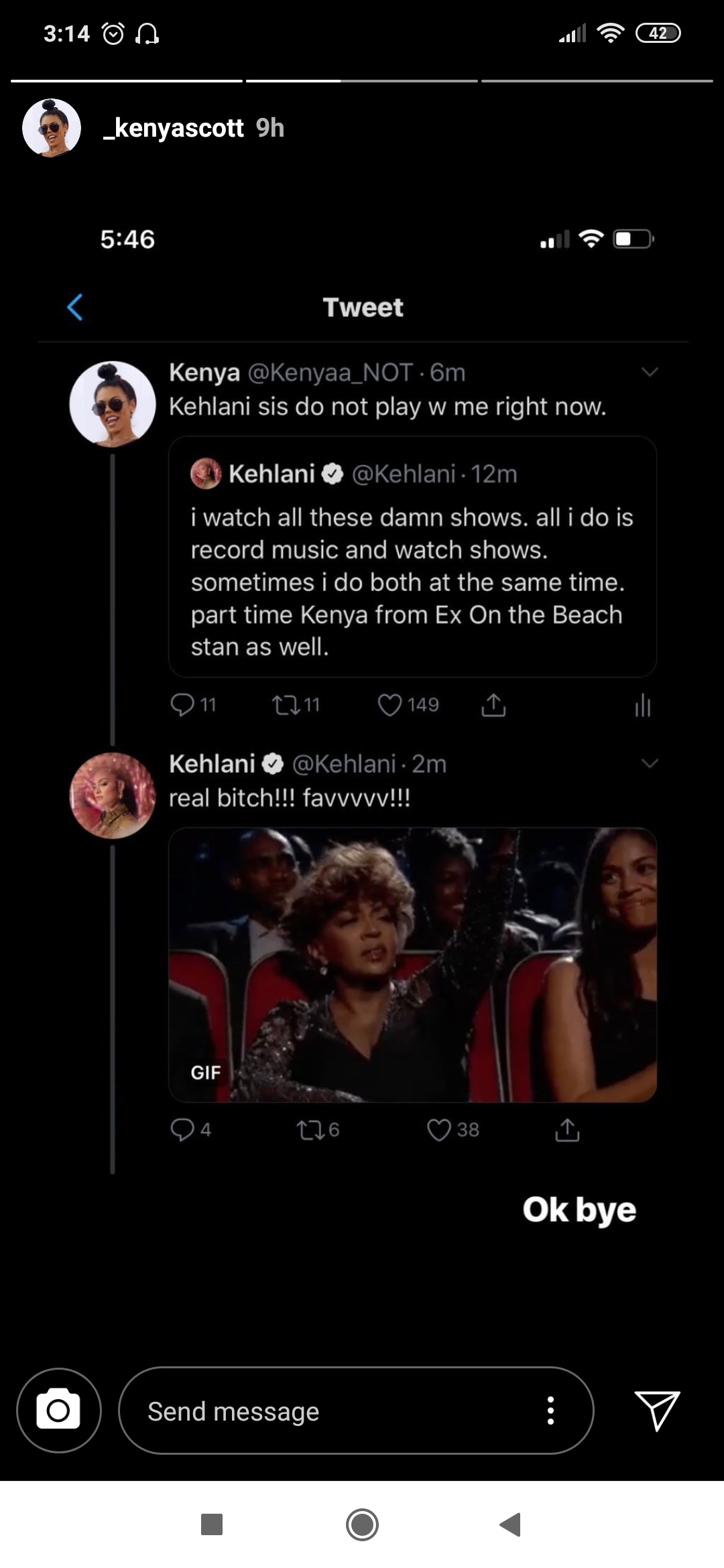A post by user @Kenya_Scouts, shared 9 hours ago on their Instagram Story, features a screenshot of a tweet. The tweet includes a chain of replies. 

The original tweet, posted by @Kenya_Underscore, reads: 

"I watch all these damn shows. All I do is record music and watch shows. Sometimes I do both at the same time. Part-time Kenya from Eggs on the Beach stan as well."

In response to this tweet, the person, likely referring to themselves as Kenya, replies with:
"Do not play with me right now."

Additionally, the screenshot includes a separate post by user @Bitch_Fave, showcasing a meme with an image and a text overlay. The caption at the bottom of this meme humorously states:
"Ok bye."